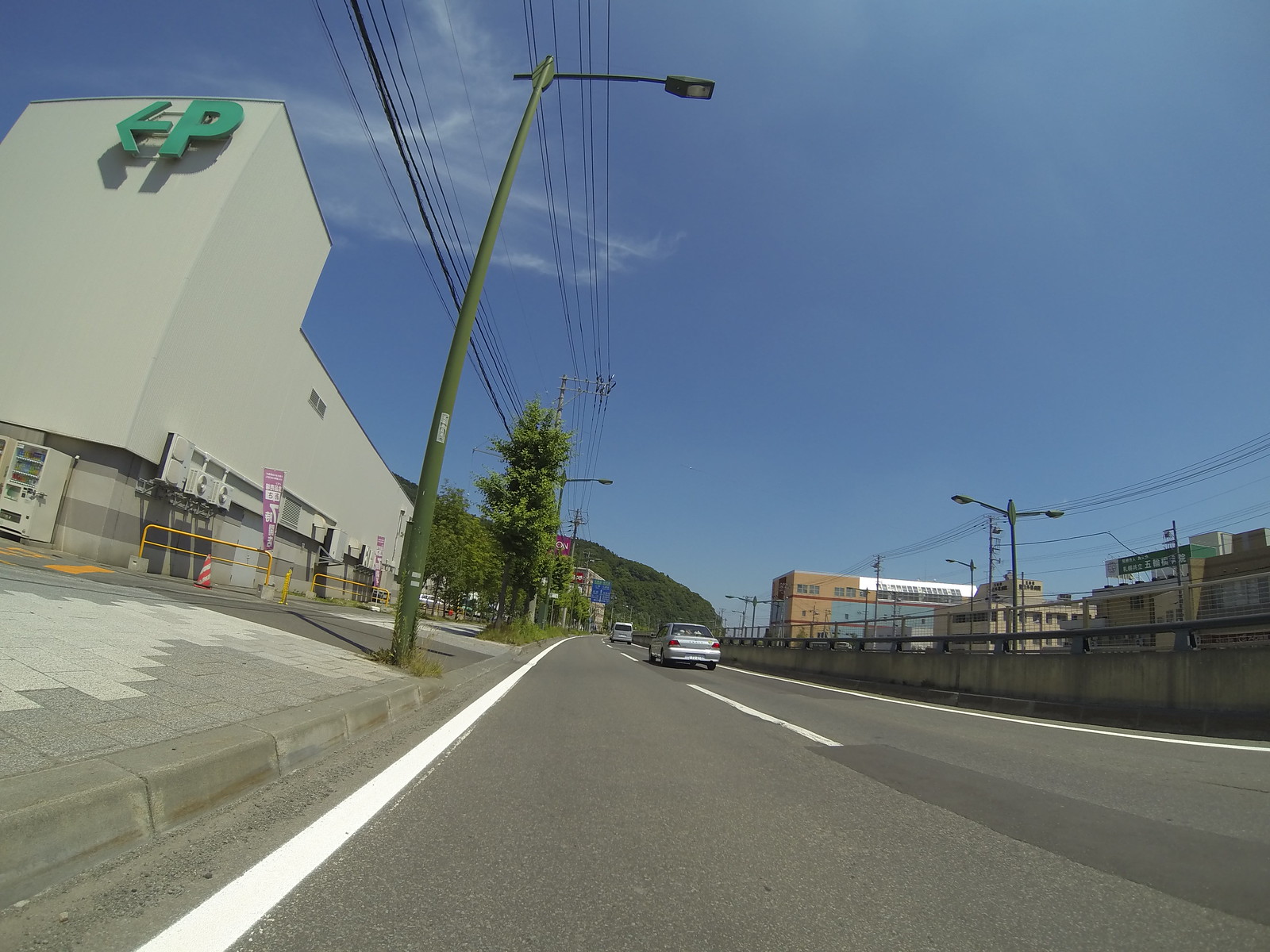The photograph captures a urban street scene from a ground-level perspective in the left-hand lane of a two-lane road, possibly indicating a one-way street given the positioning and direction of the cars. The road is asphalt with a broken white line down the center and white lines on either side. On the right side of the road, two cars—a gray sedan and a gray van—are visible, traveling in the opposite direction.

To the left of the image is a wide sidewalk adjacent to a large tan building, featuring a green capital "P" with an arrow pointing left, likely indicating a parking area. The building has an industrial feel, reflected by warehouse-like structures with fans and guardrails observed in the distance. A dark green street light and vertical metal pole are positioned near the front of the building.

The sky is a vibrant blue with few clouds, suggesting it is midday with the sun high overhead, casting pronounced shadows. Overall, the scene depicts a relatively calm city street, flanked by industrial buildings and illuminated by clear, bright sunshine.